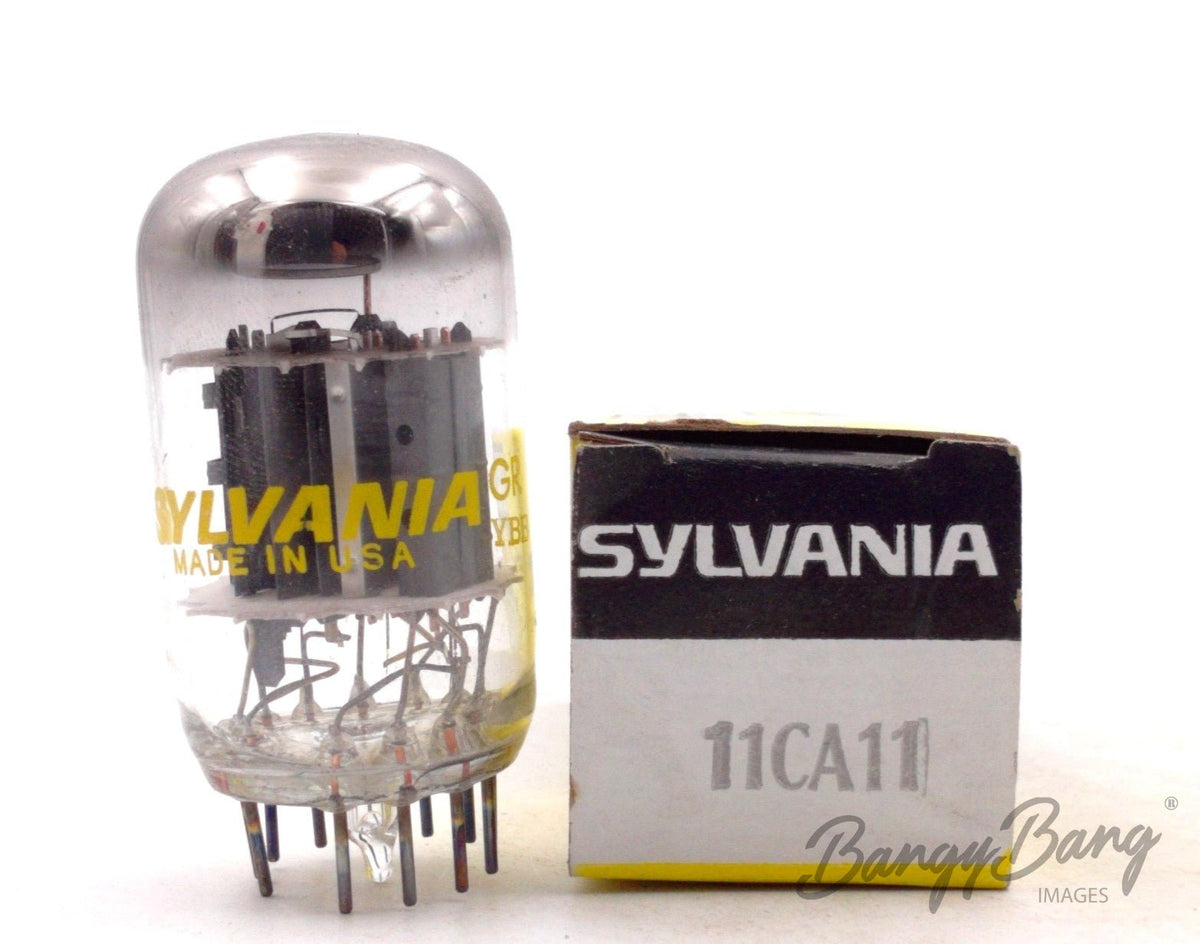The image depicts two objects on a marbleized cream table. On the left, there is a cylindrical glass fuse with a rounded, bulbous top, and several metallic prongs or pegs at the bottom, resembling an old-fashioned light bulb. The glass casing allows visibility of the internal dark gray to black components, which likely contribute to its function. The fuse is clearly branded with "Sylvania" in yellow lettering and marked "Made in the USA." To the right stands a small square box with a black top section featuring "Sylvania" in bold white letters, and a white bottom section inscribed with the identification code "11CA11" in gray. A thin yellow stripe decorates the bottom of the box, which has an open lid. The overall palette of the items includes black, white, gray, and yellow. A watermark reading "Bangy Bang Images" is located at the bottom right corner of the photograph. The items seem to be vintage electronics from the Sylvania brand.